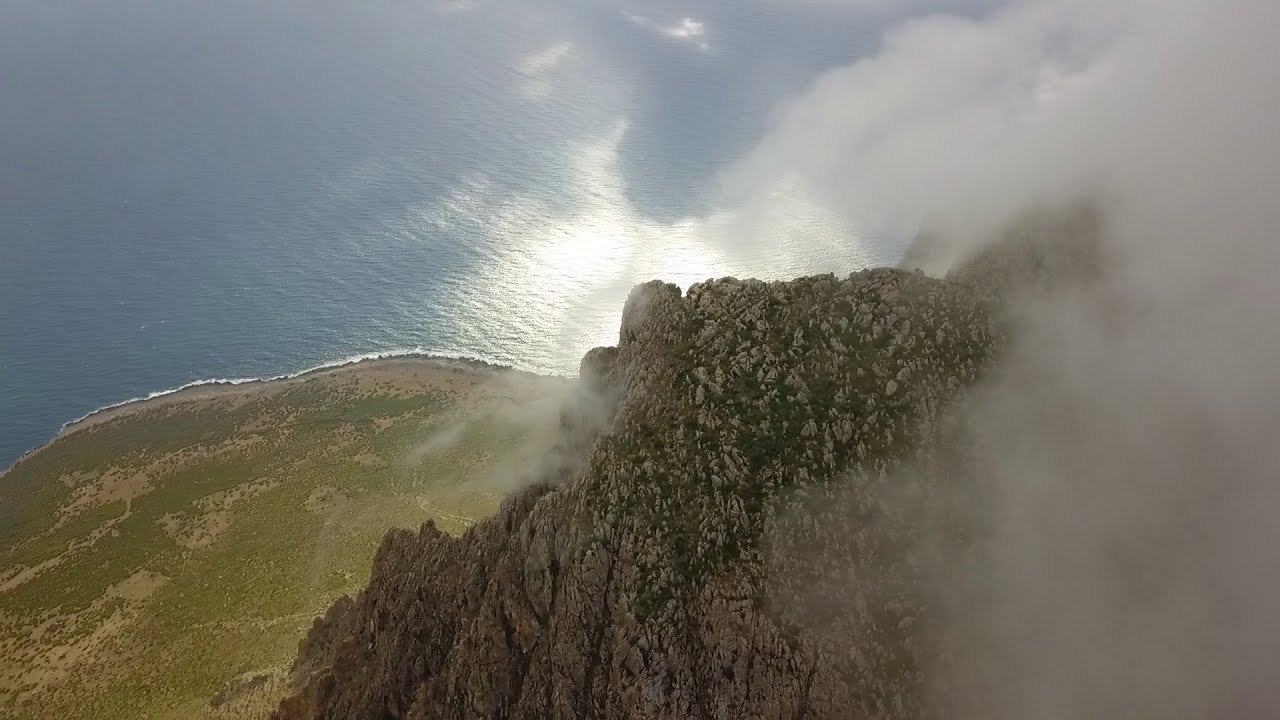The image captures a stunning aerial view, possibly taken from a drone or helicopter, showcasing a rugged cliff with rocks and sparse vegetation. The cliff is situated to the right, partially cloaked in a mist of clouds and fog, which adds a mysterious and ethereal quality to the scene. The lower half of the image depicts an open field with patches of green grass and some yellowing areas, gradually transitioning into dirt and eventually leading to a distant coastline. The coastline features a beach area and merges with the deep, bluish ocean that spans the upper left part of the image. The water glistens with calm ripples under the sunlight, reflecting a serene dark blue hue. The elevation is so high that it offers a bird's eye view of the landscape, emphasizing the sheer height and expansive view of the cliff, the stretching ocean, and the surrounding terrain. The scene is a beautiful blend of nature's elements with shades of blue, white, green, brown, yellow, and gray creating a picturesque and compelling vista.